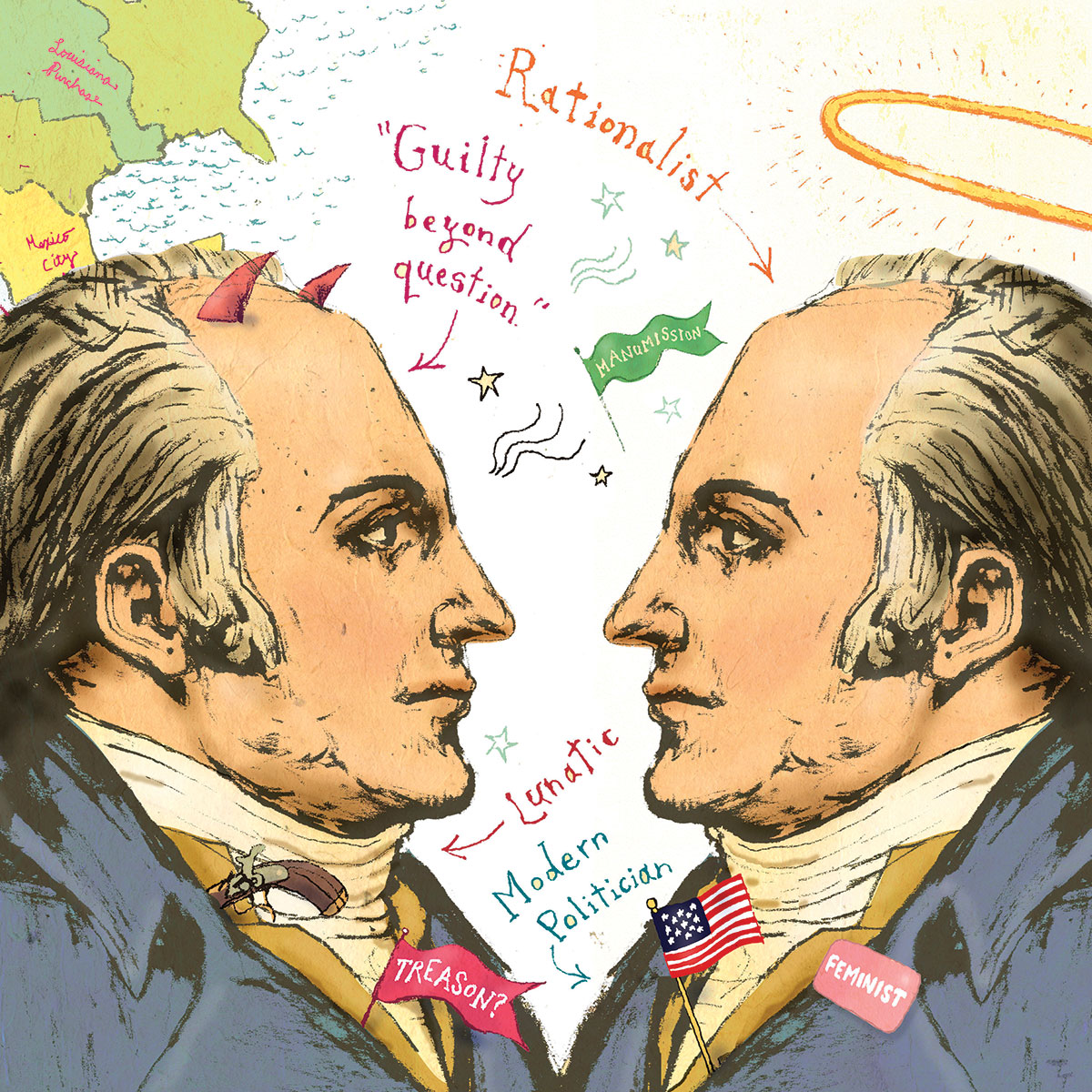The editorial cartoon portrays two identical men facing each other, illustrated in a style reminiscent of 18th-century American attire. Both men have blonde hair pulled back, long noses, long chins, sloped foreheads, and are dressed in blue coats over yellow jackets, with high-necked white shirts. The man on the left sports red devil horns and has an array of labels and symbols: "Guilty Beyond Question" in red text points to him, a red flag with "Treason?" is tucked into his collar, along with a small gun, and "Lunatic" is labeled at the bottom in red. Conversely, the man on the right is adorned with an angel's halo and is labeled "Rationalist" in orange text. He has an American flag on his chest with the word "Feminist" written in pink, and "Modern Politician" in green at the bottom. A green flag with unreadable text is situated closer to the right figure. The background includes a map in the upper left corner, with portions labeled "Mexico City" at the bottom and "Louisiana Purchase" in the middle, surrounded by star symbols and water waves, while the rest of the background remains largely white.